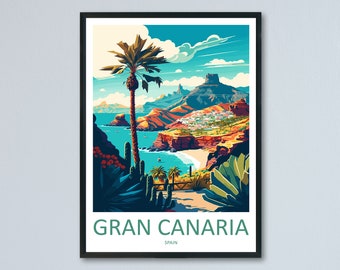The image is a perfectly square photograph set against a light gray background. At the center of the composition, a thin black-framed picture is prominently featured. Encased within the frame, a white matting provides a crisp border that accentuates the artwork at its core. At the bottom of the matting, the text "GRAN CANARIA" is elegantly displayed in all capital letters, rendered in a teal hue. Below this text, in much smaller print, lies the word "Spain," though its diminutive size renders it somewhat difficult to read. The artwork itself is a picturesque depiction—possibly a drawing or painting—of an outdoor scene on Grand Canaria. It showcases a tranquil setting with a tall palm tree reaching towards a blue sky dotted with scattered clouds. A serene body of water graces the scene, accompanied by various plants and lush greenery, culminating in a small stretch of land. This framed piece of art, celebrating the scenic beauty of Grand Canaria in Spain, hangs solitary on the gray wall, with no human presence to distract from its serene and captivating imagery.